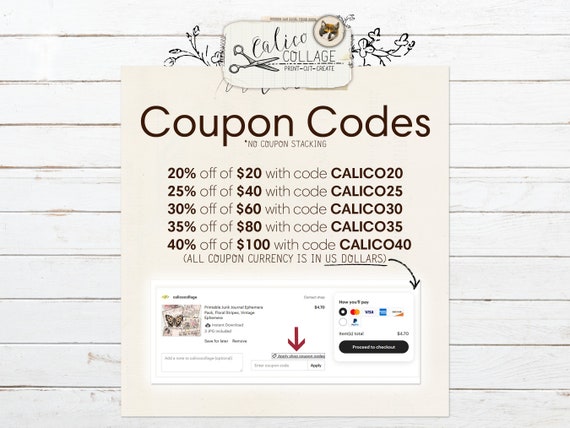The image features an advertisement against what appears to be the white, horizontally-slatted wooden siding of a building. The advertisement itself resembles a piece of paper affixed to the siding. The main focus is on various coupon codes for "Calico Collage," a service emphasizing print, cut, and create activities, and highlights a logo featuring a pair of scissors above the words "Calico Collage," with an illustrated calico cat and floral background.

Prominently, the ad lists several discount coupon codes, stipulating no coupon stacking, with the following details:

- 20% off on purchases of $20 with code Calico20
- 25% off on purchases of $40 with code Calico25
- 30% off on purchases of $60 with code Calico30
- 35% off on purchases of $80 with code Calico35
- 40% off on purchases of $100 with code Calico40

All the discounts are in US dollars. 

Below the list of coupon codes, an arrow points downward to a section regarding payment methods, which appears blurry and difficult to decipher but implies options like Visa and American Express. The background gives a contrasting look of lined paper, with some lines appearing hand-drawn in pencil, enhancing the crafted aesthetic. Finally, an instruction mentions that the cost to download these coupons is $4.90 and suggests ways to pay for them, tying the visual and textual elements together cohesively.